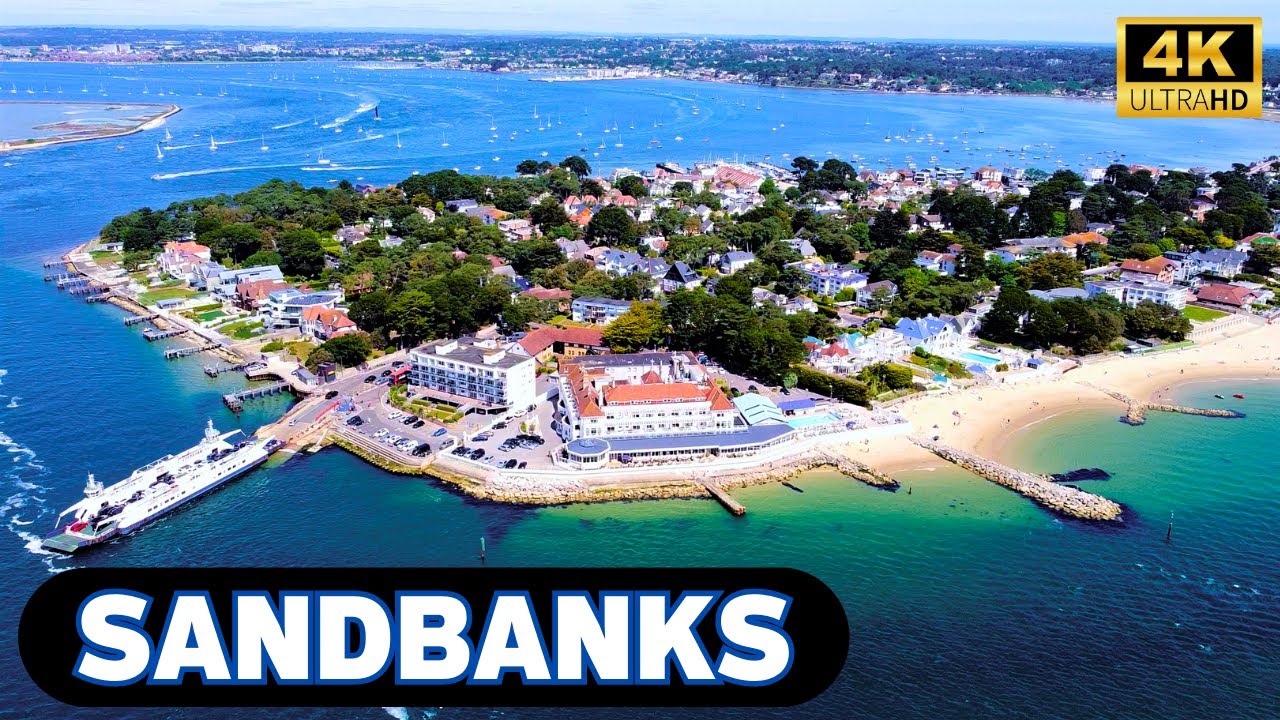This vibrant 4K Ultra HD image captures a stunning sandbank projecting into the ocean, surrounded by water on three sides. At the bottom left of the image, the text "Sandbanks" is displayed in bold white over a black background. The upper right corner features the "4K Ultra HD" label in black text on a gold background. The sandbank is adorned with an array of white buildings with tan roofs, including resort houses, mansions, and larger structures, interspersed with lush trees. Several piers extend into the vivid blue and green ocean, where multiple boats are docked. On the lower left side of the image, a cruise ship is seen docking at an outcropping near a parking lot adjacent to a larger building. Additional boats dot the waters around the sandbank, with more land and buildings visible in the distance, enhancing the image's sense of depth and detail.